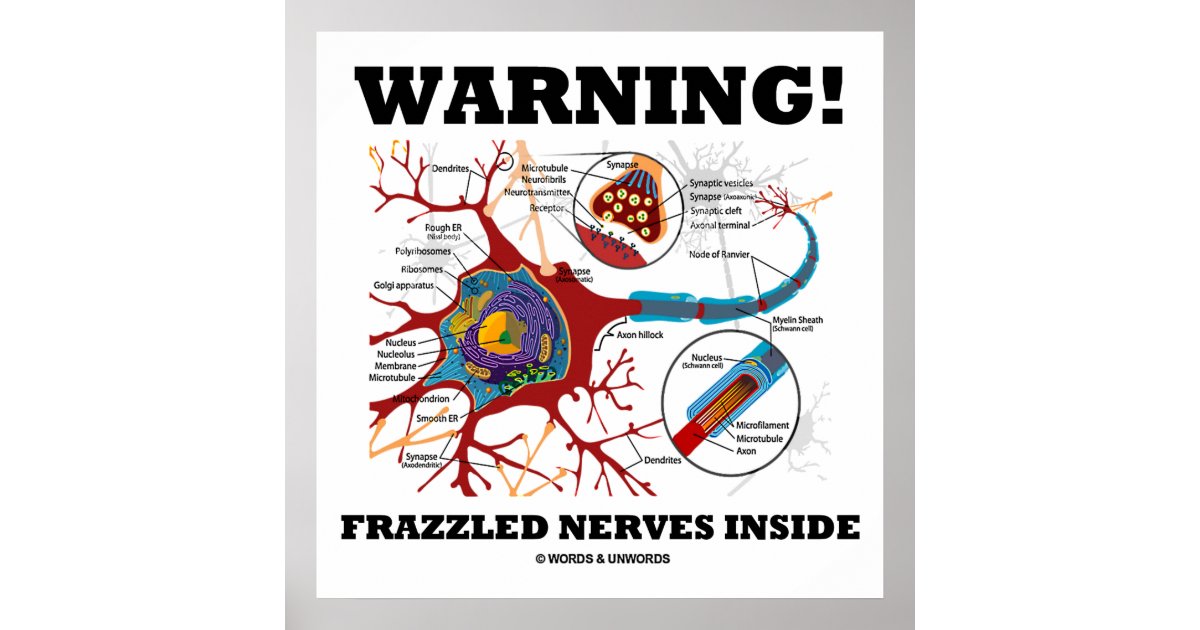The image is a scientific poster featuring a detailed diagram of the nervous system. It has a solid gray border with a light blue background surrounding a central white box. At the top of the white box, in large, bold, black, all-caps text, the word "WARNING" is prominently displayed next to an exclamation mark. Below this, the phrase "FRAZZLED NERVES INSIDE" is written in bold black text, though not as large as the warning.

The main illustration depicts nerves inside the body, with the nerves shown in burgundy and highlighted by blue areas that encapsulate them. The diagram includes various magnified sections and detailed annotations, labeling parts such as dendrites, rough ER, polyribosomes, ribosomes, Golgi apparatus, nucleus, nucleolus, membrane, microtubule, smooth ER, synapse, axon hillock, myelin sheath, synaptic vesicles, synaptic cleft, axonal terminal, and node of Ranvier. Arrows and smaller images further emphasize and clarify specific aspects of the nervous system. The overall presentation combines the intricate detail of nerve anatomy with clear text descriptions to educate the viewer about the structure and function of nerves.